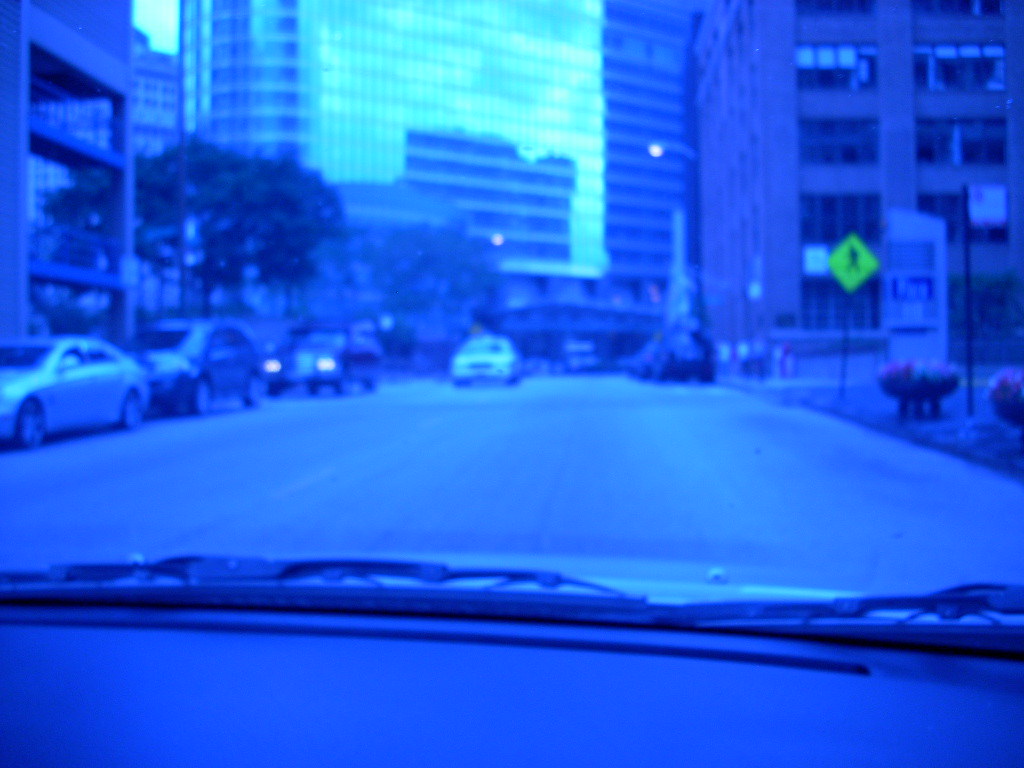The photograph, possibly taken from the passenger side of a car, captures an urban scene in a large city. The image is tinted heavily purple, an artificial adjustment that colors everything—including the cars, roads, and dashboard—in a distinct purple hue. The perspective is first-person, looking out over a paved road with double yellow lines from inside the vehicle. Prominent in the center of the image is a tall, skyscraper-like building with reflective glass windows. On the right, there's another towering structure and a yellow pedestrian crosswalk sign. To the left, there's a multi-level parking structure and a line of cars waiting to turn, including some parked vehicles and a police car heading towards the driver. The dashboard is minimally visible, with black surfaces and windshield wipers in sight. The photo, which has a somewhat blurry and filtered quality, also shows the mirrored reflection of the sky on the skyscraper directly ahead, adding a surreal depth to the overall composition.